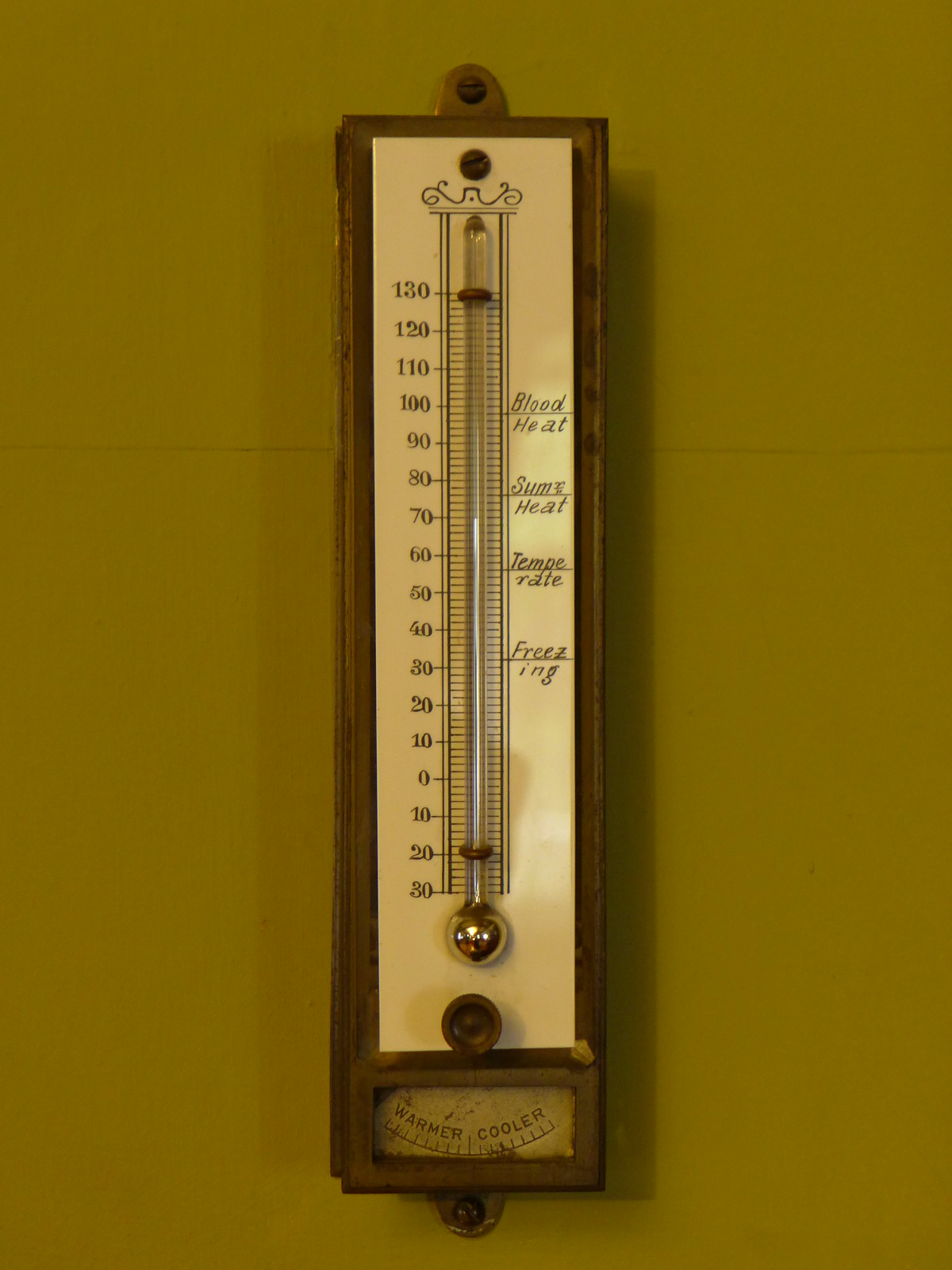The image features an antique Fahrenheit thermometer encased in a wooden frame with a brass plaque engraved with numbers ranging from -30 to 130 degrees. The thermometer, currently reading 69 degrees, has various descriptive terms inscribed in cursive along its side. At 32 degrees, the marking reads "freezing." Further up, at 56 degrees, it reads "temperate," and at 98 degrees, "blood heat" is noted. The marking at 76 degrees is partially illegible, beginning with the letter "S" and indicating some level of heat. This intricate, vintage piece embodies both functional and aesthetic historical charm.